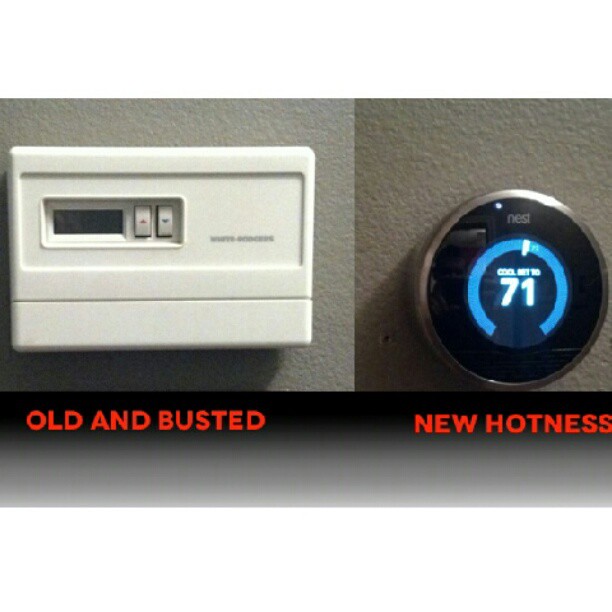This image is a digitally created graphic, blending two distinct photographs. The left side features an old-style household thermostat, slightly larger than the element on the right. This vintage thermostat is a white rectangle with a gray digital display, showing simple red and blue arrows for increasing and decreasing the temperature, respectively.  

The right side displays a smaller and darker image of a modern Nest thermostat. The Nest device is round with a sleek black face, showcasing a digital screen that includes a blue circle and the text "Cool" followed by "71," indicating a set temperature of 71 degrees Fahrenheit. 

Below the combined images, there is a gradient black background. Accompanying text labels the thermostats: "Old and Busted" in red beneath the vintage model, and "New Hotness" in black and red beneath the Nest thermostat.